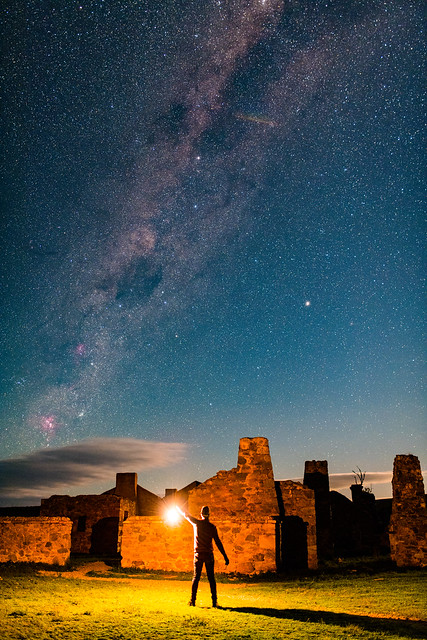This nighttime image captures a stunning scene under a twilight sky that transitions seamlessly into an expansive, star-filled canvas. The deep blue backdrop is scattered with countless stars, forming a mesmerizing view of the Milky Way, which appears as a dense cluster of stars stretching from the horizon upward. In the sky, near the left, a purplish-pink cloud extends into the middle of the frame, adding a dramatic touch to the celestial display.

Below this breathtaking sky, the bottom half of the image presents the ruins of an ancient stone brick house, now largely dilapidated with crumbling walls. A lone figure, standing in a field of green grass near the ruins, holds up a bright light, illuminating the surroundings with a white glow. This person faces the ruins, their arm extended forward, perhaps suggesting exploration or discovery. The yellow-toned ground below contrasts vividly with the blue and pink hues above, creating a striking artistic composition that juxtaposes the tiny human figure against the vast, awe-inspiring night sky.